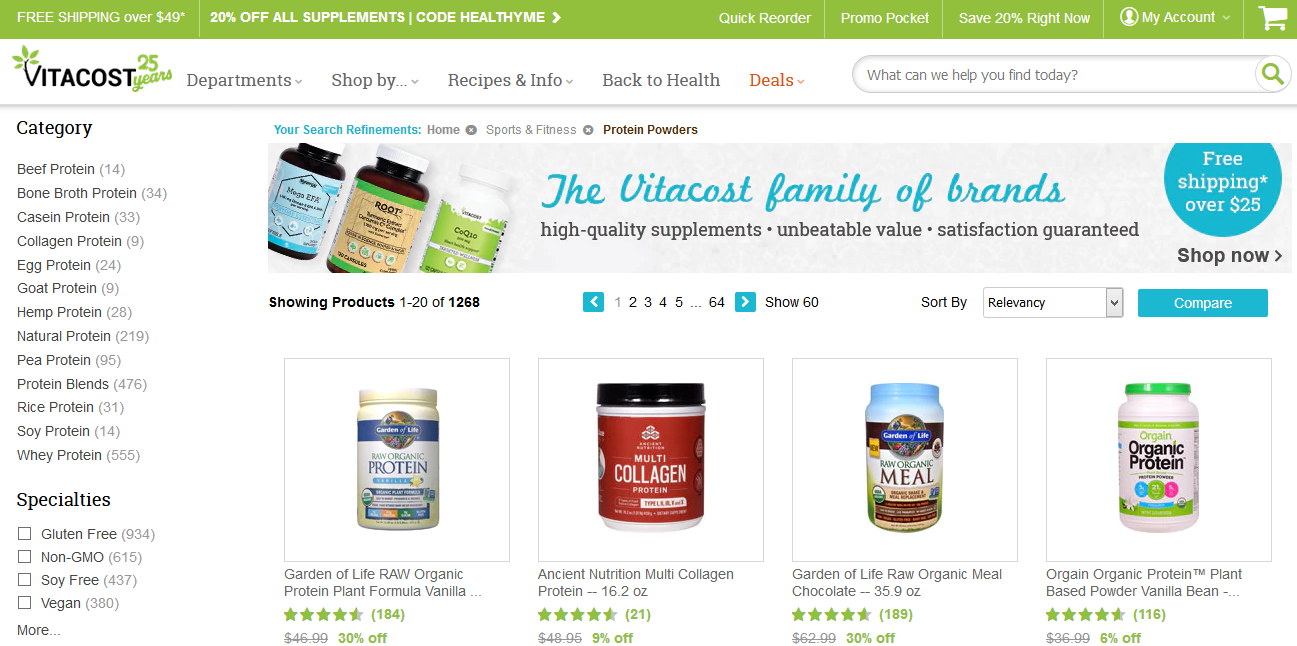This image captures the homepage of the VitaCost website. In the upper left corner, the VitaCost logo is prominently displayed, featuring a stylized "V" encircled by plant-like leaves on its left side, symbolizing natural and health-focused products. A green bar at the top of the page highlights several promotional elements: "Free shipping on orders over $49" on the left, and "20% off all supplements" with the promo code "HEALTHYME" on the right.

Just below this bar, there's a quick reorder promotion promising an additional 20% savings. To the right, the navigation menu includes options for "My Account" and "Shopping Cart."

The main website navigation is organized horizontally underneath, with categories such as "Departments," "Shop By," "Recipes & Info," "Back to Health," and "Deals." A search bar is positioned just below this main menu for easy access.

On the left-hand side of the page runs a vertical menu labeled "Categories," guiding users through various product selections. Beneath this, there's another menu labeled "Specialists," likely offering specific recommendations or featured products.